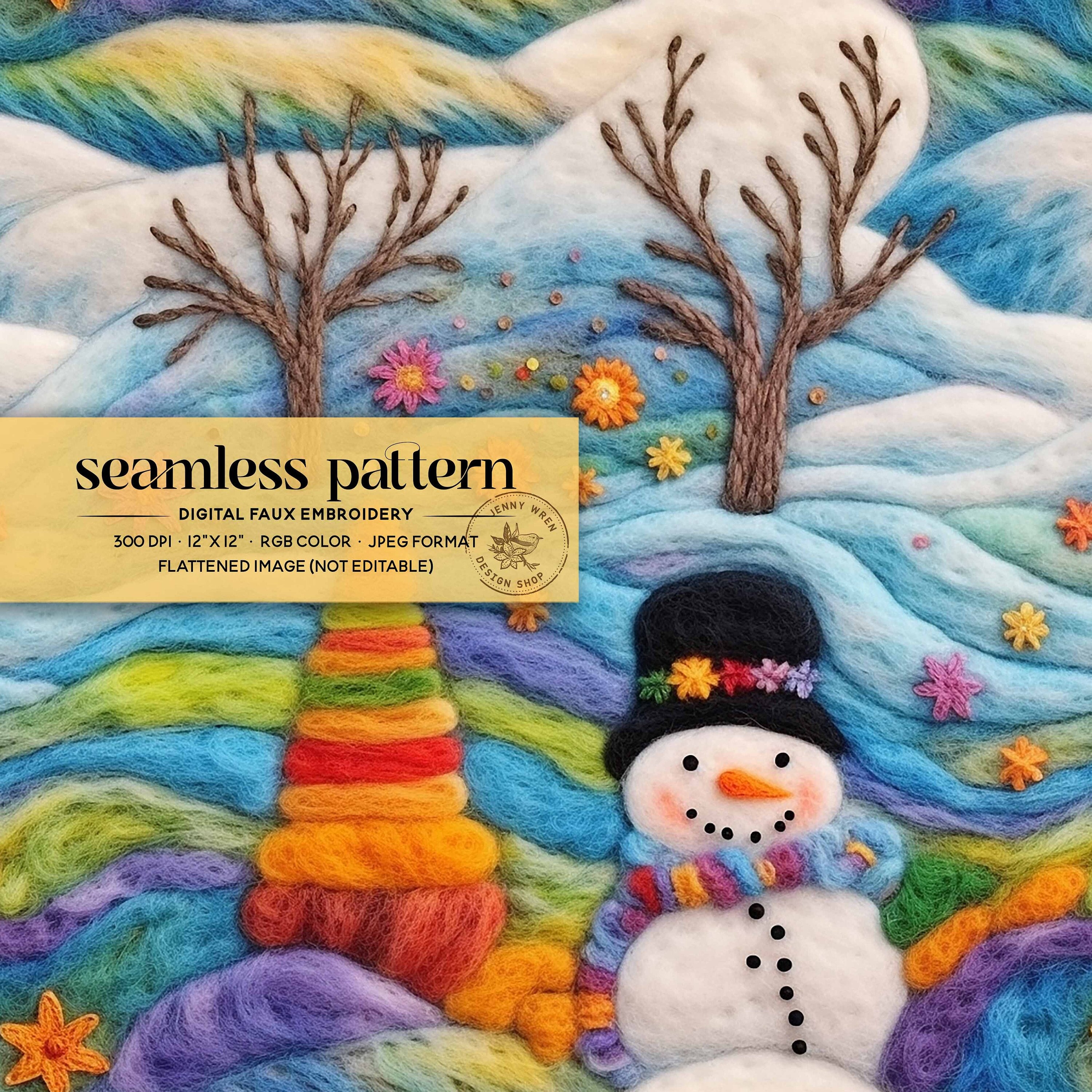This detailed image showcases an advertisement for a digital faux embroidery design, specifically a seamless pattern by Jenny Ren Design Shop. The scene is a vibrant, colorful winter landscape crafted out of felt with meticulous embroidery details. At the upper part of the image, yellow-capped rolling hills and blue clouds or possibly snow create a textured and rich background. Situated in the upper middle are two bare brown trees, surrounded by bright flowers without stems. The felt landscape features a wintry snowman prominently positioned at the bottom right. The snowman has intricate details including black button eyes, a carrot nose pointing to the right, a dotted black mouth, and a series of black dots down its snow-white body. It wears a black hat adorned with a floral wreath and a multi-colored scarf with purple, orange, magenta, and blue hues.

The entire scene is framed by horizontal, curved lines of multicolored felt, adding a whimsical and textural depth to the composition. Additionally, there is a yellow, transparent banner on the middle left side of the image that contains important text details: "Seamless Pattern," "Digital Faux Embroidery," "300 DPI," "12 inch by 12 inch RGB color JPEG format," and "Flattened Image Not Editable." The banner is accentuated with a stamp that reads "Jenny Ren Design Shop," illustrated with a flower and a bird. The image itself is in a square format, emphasizing the detailed combination of felt textures and vibrant colors in this unique embroidery design.